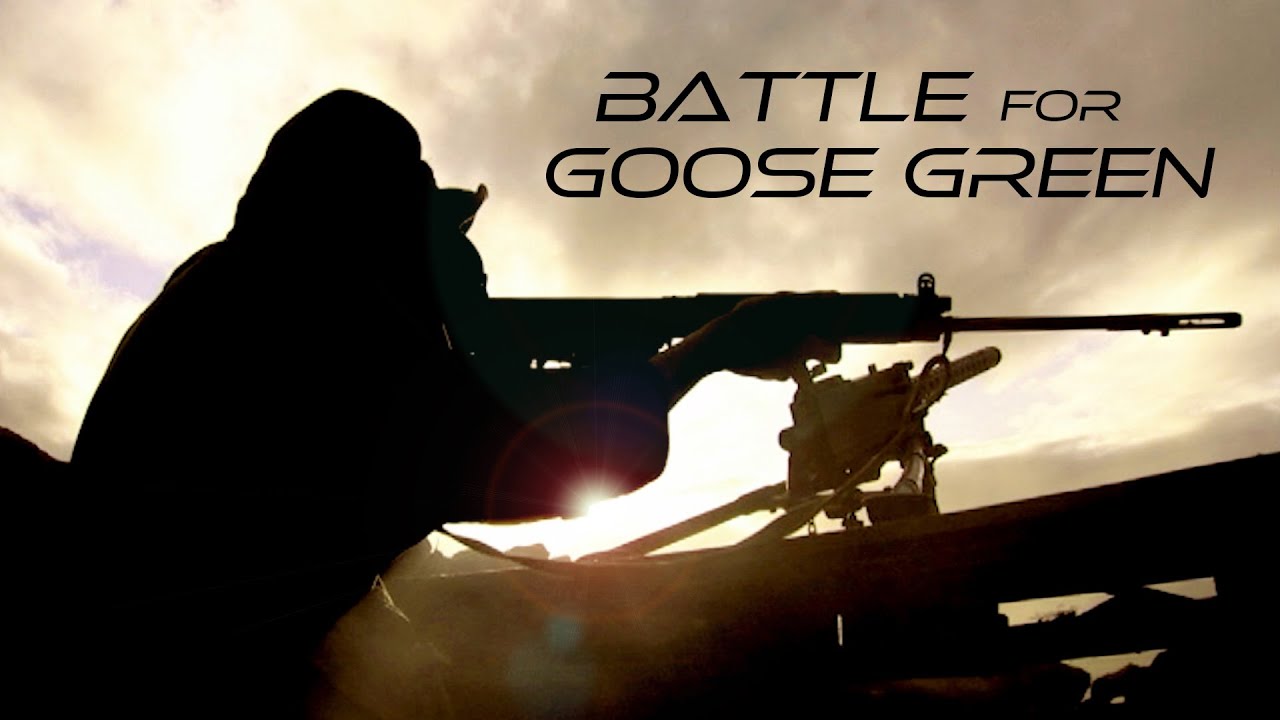The image is a dramatic and intense poster titled "Battle for Goose Green," written in two rows of black letters at the top right. Dominating the left side is the black silhouette of a person holding a long-range firearm, complete with a scope, aimed to the left of the frame. Their figure is stark against a cloudy, overcast sky, which, despite its purplish-gray haze, reveals it is daytime due to a visible sunbeam piercing through below the person's arms. To the left of this silhouette, a machine gun is mounted on a wooden barricade structure, suggesting a war or battle scenario. The overall imagery evokes a sense of imminent conflict, possibly hinting at a video game or movie sequel set in the tense backdrop of Goose Green.